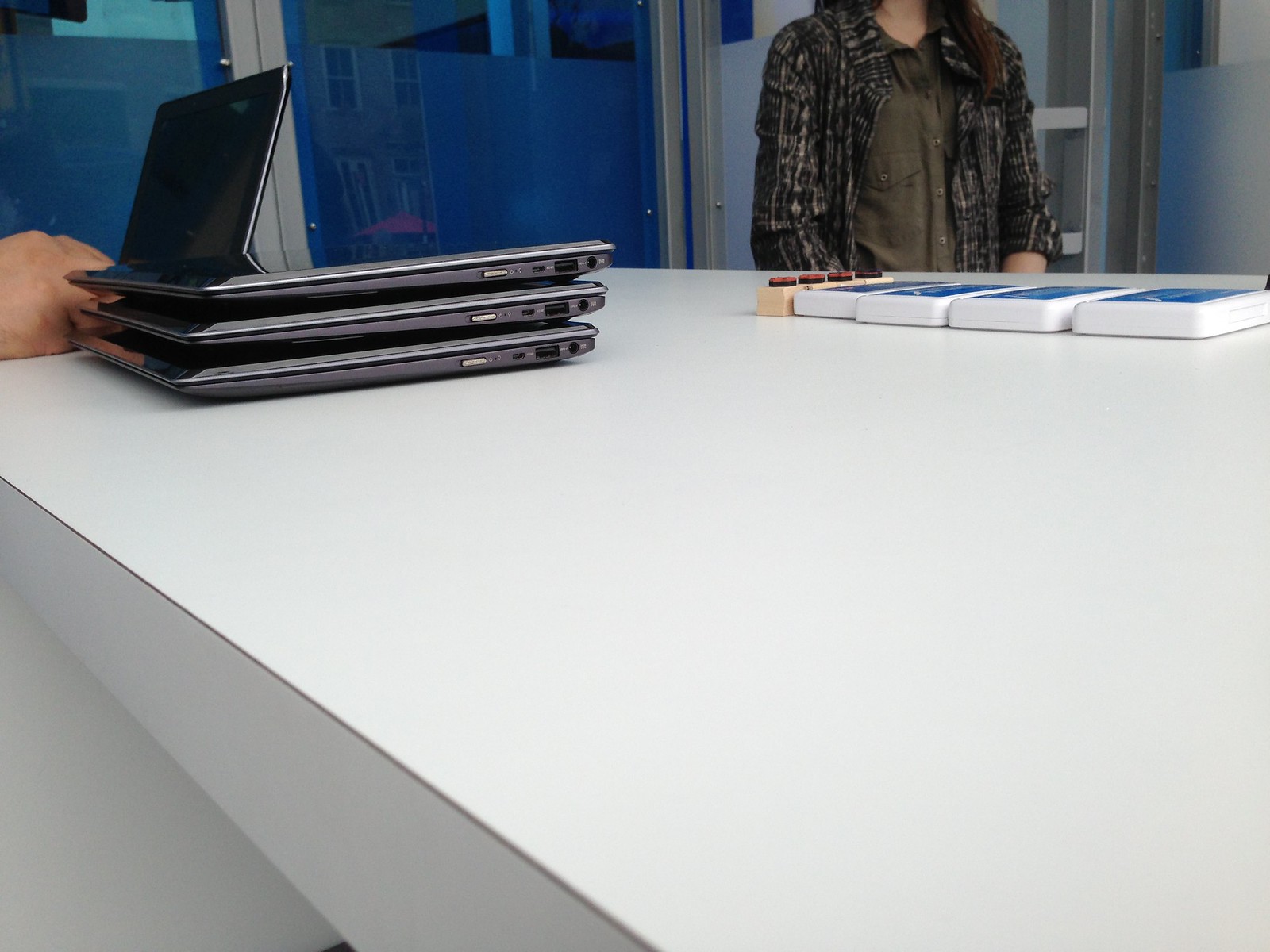In this indoor photograph, taken from a low angle as if from someone seated at a table, the foreground features a large white desk. On the left side of the desk, three laptops are stacked on top of each other, with the top one having an object sticking out as if to hold it up. To the right of the laptops, there are four white objects with blue tops, neatly lined up next to each other, accompanied by a beige rectangular object with four red buttons on top. The surface close to the viewer is clear.

In the background, a woman is visible from her shoulders to her waist, dressed in a brown jacket over a greenish shirt. In the further background, there is a blue door with metallic frames separating its window panels. Additionally, a hand, possibly from another person, is seen on the left side of the image. The overall scene captures an organized yet busy workspace within a building setting.